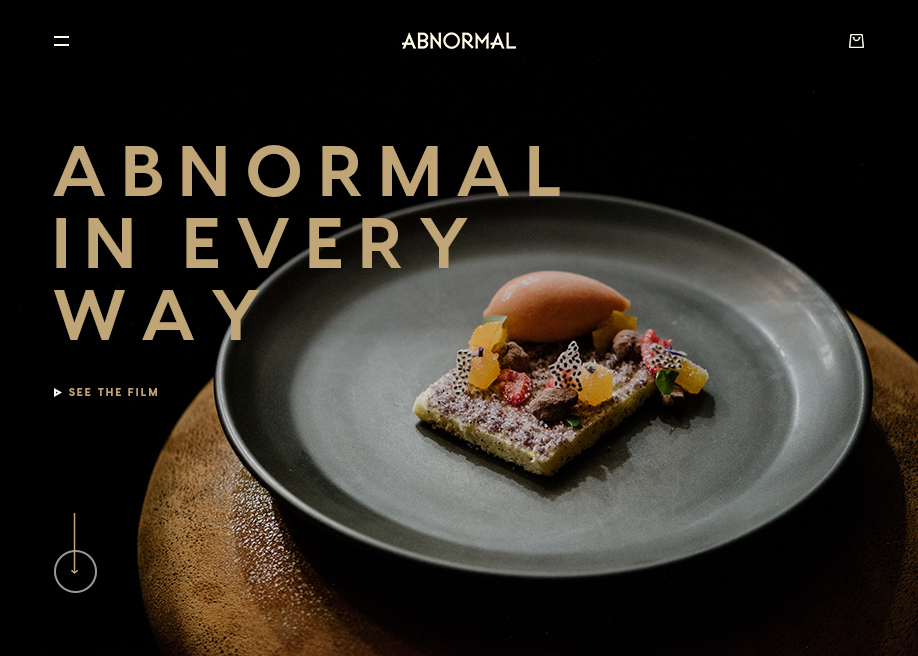The advertisement features a sleek, minimalistic design with a focus on contrast and texture. The background is entirely black, creating a striking canvas for the elements that follow. In the top left corner, there are two lines resembling a minimalist menu icon. The word "ABNORMAL" stands out prominently in the center of the page, rendered in a sleek tan or white font. Just to the right, a white shopping bag icon is present, hinting at the theme of shopping or e-commerce.

In the center of the image, a silver plate takes the stage, showcasing a tantalizing dish. The plate holds a beautifully presented waffle adorned with possible sugar and cinnamon. The waffle is garnished with chia seeds, adding a healthful touch, and vibrant raspberries that add a burst of color. There are also cubes of an unidentified ingredient that resemble ginger, and an elongated, egg-like object that intriguingly resembles a sweet potato.

The silver plate rests atop a striking piece of stoneware or pottery. This base is a brown, tannish color with a porous texture, highlighting shades of dark brown and black within its surface. The plate and the stoneware are only partially visible, with about three-quarters of the stoneware's round form displayed, the remainder cut off by the corner of the image.

Dominating the lower portion of the advertisement is the bold tagline "ABNORMAL IN EVERY WAY" in all caps, written in a dark tan font. Nearby, a white right triangle points towards the call to action in capitalized dark tan letters, "SEE THE FILM." Below this, a white circle features a tan arrow stretching from the top to the center, guiding the viewer’s eye towards the core message of the advertisement.

Overall, the detailed composition, contrasting colors, and intriguing dish emphasize a sophisticated yet curious allure, drawing viewers into the advertised content.